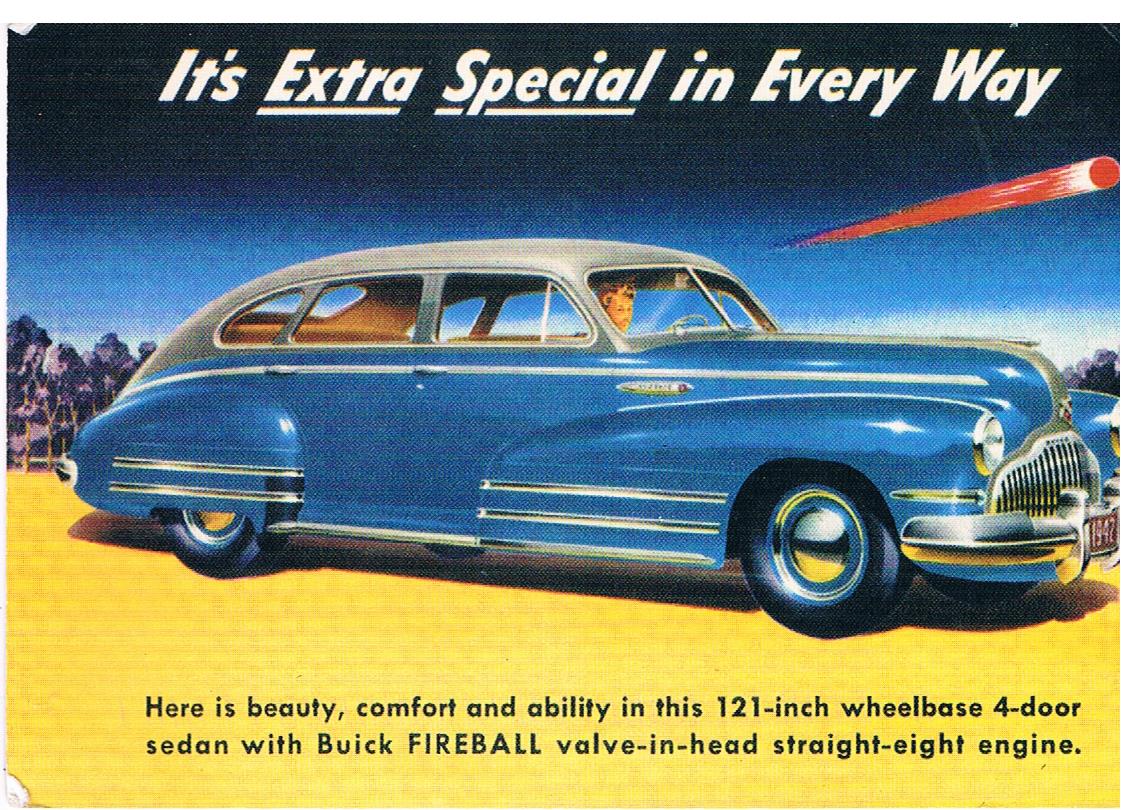The advertisement is a horizontal scan of an old magazine ad featuring a striking 1950s-style sports car. At the top, in white letters, the slogan "It's extra special in every way" is prominently displayed, with "extra special" underlined for emphasis. Below, the main visual showcases a large, blue four-door sedan with chrome wheels and a silver roof, elegantly framed with white stripes near the wheel wells. The car sits on a yellow surface, in front of a background featuring purple-looking trees and a blue-to-black gradient night sky that suggests a transition from day to dusk. Adding to the dramatic night scene, a red meteor—symbolizing the Buick Fireball valve-in-head straight-8 engine—streaks through the sky. At the bottom, black text details the features of the car: "Here is beauty, comfort, and ability in this 121-inch wheelbase 4-door sedan with Buick Fireball valve-in-head straight-8 engine," effectively linking the imagery of speed and power with the vehicle's technical attributes.